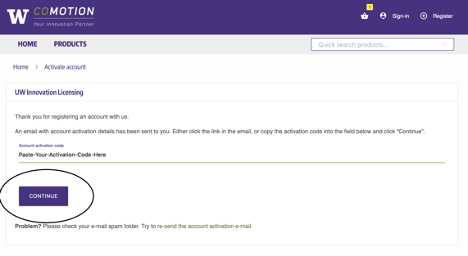The image features a user interface with various elements organized in a structured layout. 

At the top of the image, there's a dark purple border. On the top-left corner within this border, the text "W Commotion - Your Innovation Partner" is partially visible but slightly blurry. 

On the top-right corner, there's a shopping basket icon accompanied by a generic default profile picture. Next to these icons, there are two buttons labeled "Sign In" and "Register."

Below this top section, a light purple box extends across the width of the image. On the left side of this light purple box, there are navigation links labeled "Home" and "Products." To the right of these links, there's a search box labeled "Quick Search Products." 

Underneath the light purple box, there's another section of text. On the left side, it reads "Home Activate a Core" (though the exact wording for "Core" is uncertain due to blurriness). Below this, it says "UW Innovation Licensing."

Further down, there's a message thanking the user for registering an account. The message explains that an email containing account activation details has been sent to the user. It instructs users to either click the link in the email or copy the activation code into the field below and then click "Continue."

At the bottom of this section, there's a prompt for users to paste their app activation code. Adjacent to this field, there's a purple rectangle button labeled "Continue," which is notably encircled by a black, hand-drawn circle.